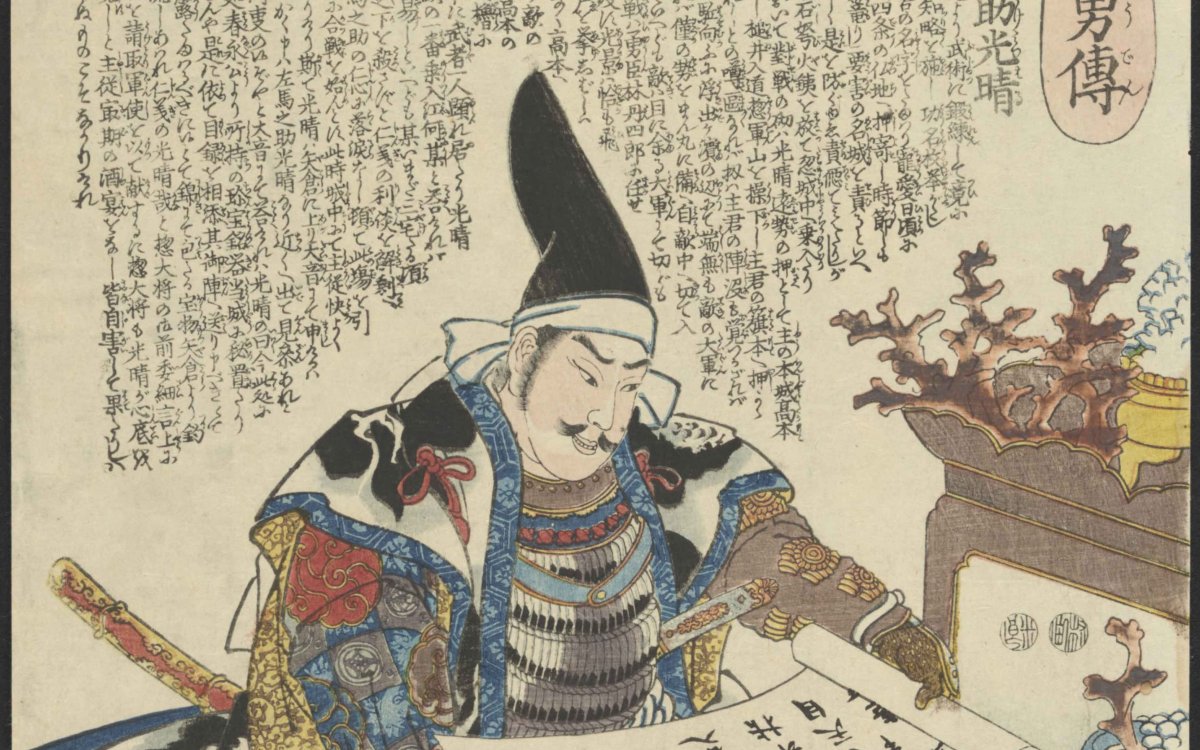The image depicts an ancient and detailed painting, likely of East Asian origin, either Japanese or Chinese, showcasing a central figure who holds a commanding presence. The man, appearing heavyset with a distinctive black mustache and sideburns, dons an elaborate and colorful kimono. His attire is adorned with intricate floral designs in hues of red, blue, and white, further complemented by a samurai-style armor across his chest. A sword hilt is visible from behind him, with a dagger sheathed at his side. A tall, black peaked hat with a white cloth wrapped around his head extends about a foot above him, adding to his imposing appearance. He is intently reading from an unrolled scroll, bearing a devious smile on his face.

Surrounding the man is a cream-colored background filled with columns of black Chinese characters, prominently displayed at the top and cascading down the sides, contributing to the ancient and scholarly atmosphere of the painting. A little desk, supporting small plants or trees, is situated nearby, enhancing the scene’s intricate details. The character's coat, described as having black, blue, and white hues, possibly resembles piano keys, and features gloves embellished with gold. Additionally, the artwork hints at a fireplace-like brown object in the lower right corner, and the man’s distinctive appearance is heightened by his pointed eyebrows and the elaborate decorations on his attire, including a shawl with black spots.

Overall, the painting exudes an aura of antiquity and depth, ripe with historical and possibly mythical significance.